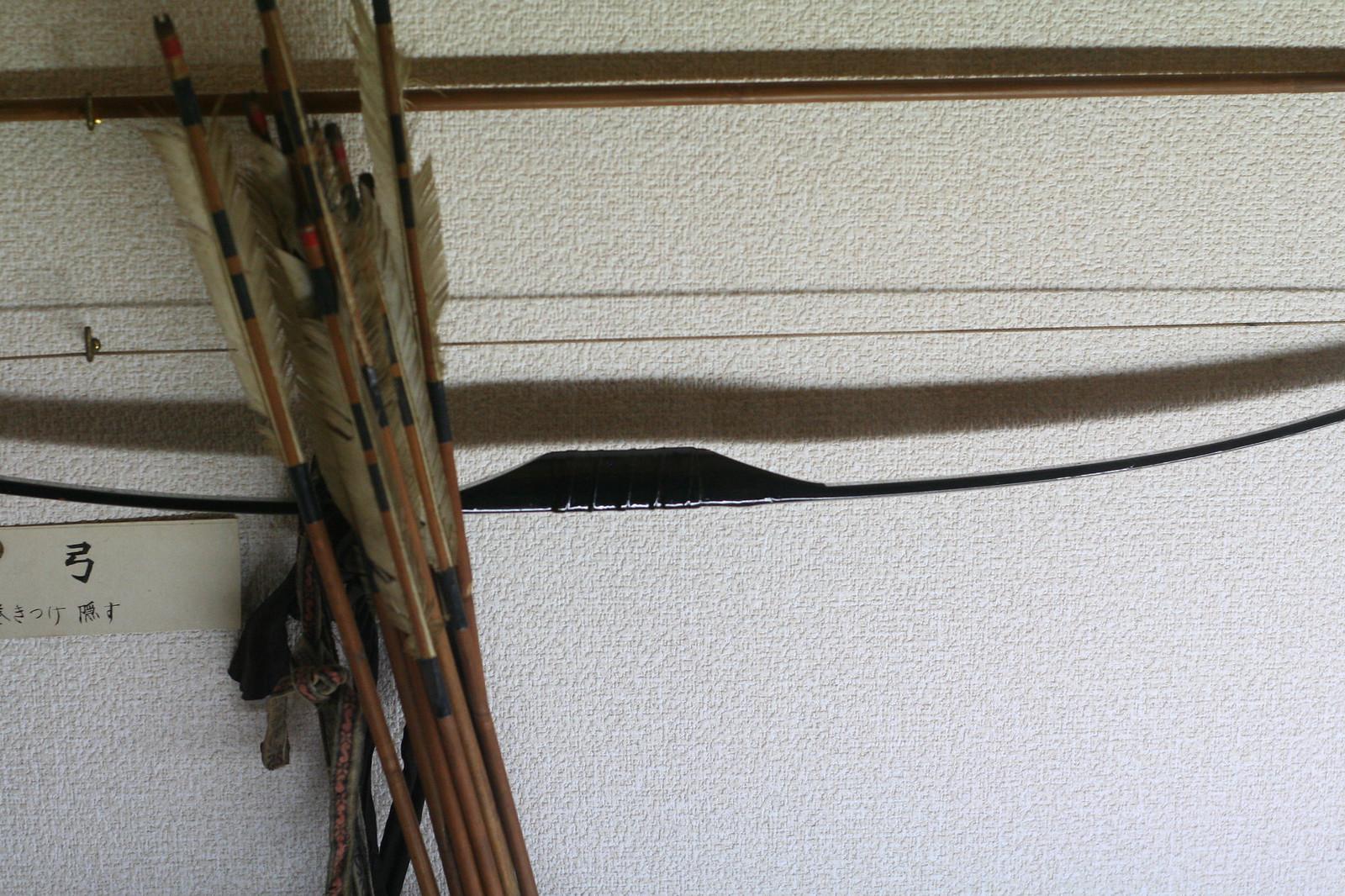This close-up color photograph captures the intricate details of several handmade arrows arranged against a textured white background. The arrows, numbering around eight, are crafted from light brown dowels or sticks, which might be wood, reed, or bamboo. Each arrow is fitted with white, off-white, and light brown feather fletching, meticulously held in place by dark black wrappings. Though the feathers add an authentic, rustic charm, some, especially on the top arrow, appear slightly frayed. To the left side of the image, beneath the arrows, there is a white label featuring Japanese kanji and hiragana characters. Above, a wooden rod runs along the top, complementing the traditional aesthetic of the arrows. The image, if rotated 90 degrees left, would make the objects more immediately recognizable as arrows.